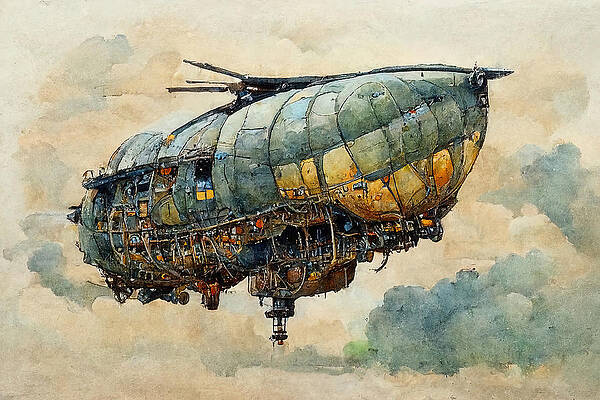In this detailed hand drawing, an intricate fantasy airship, reminiscent of both a dirigible and a blimp, soars high amidst the clouds. The large, balloon-like structure at the top features numerous vibrant colors, predominantly greens with patches of blue and sections of yellowish-orange. These colors blend together as if the airship is patched and weathered, giving it a slightly steampunk or post-apocalyptic vibe. Propellers stick out from the top, suggesting propulsion mechanisms, while the overall shape of the airship appears somewhat misshapen and worn, as though it’s been through rough conditions. 

The sides of the airship reveal multiple windows and openings, with suggestions of faces or objects peeking out, adding a sense of life and activity on board. Below the main balloon, the airship is partially shredded, with dangling strings, possibly indicating damage or an incomplete structure. Near the bottom, an observation deck or a docking tower is visible, likely a station for smaller airships or airplanes to dock.

The backdrop of the drawing feels cohesive with the airship, painted in earthy tones of tan, green, gold, and beige, adding to the aged, watercolor-like aesthetic of the scene. Overall, the fantasy airship, with its mechanical and colorful components, floats eerily suspended in the sky, enveloped in a somewhat gloomy, overcast atmosphere.